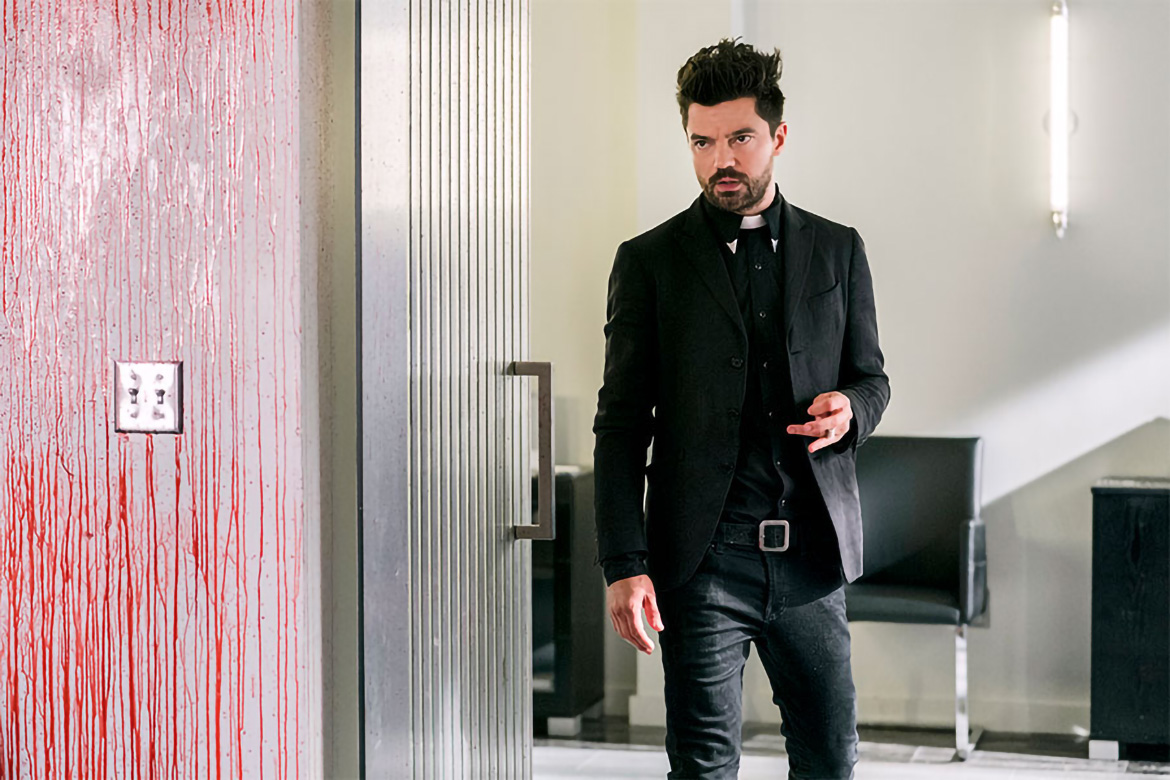In this detailed scene from the TV show *Preacher*, the actor Dominic Cooper, playing a priest, is depicted walking through a silver-plated door with a darker gray handle. Dressed in the traditional clergy attire, he wears black pants, a black jacket, and the distinctive white priest's collar at the front. His appearance includes black, somewhat messy medium-length hair, a black beard, and a mustache, alongside a light, scruffy beard. His left hand is held in front of him while his right hand rests by his side.

In the background of the room he is exiting, there is a white wall with a black leather-backed chair placed against it, along with a fluorescent tube light hanging vertically. A counter is also discernible against the wall. To the left of the doorway within the scene, another wall features pronounced red streaks that intensify near the bottom, resembling streams of blood, fitting the often dark and graphic nature of the show. A light switch is also mounted on this wall, adding to the detailed environment depicted in the image.